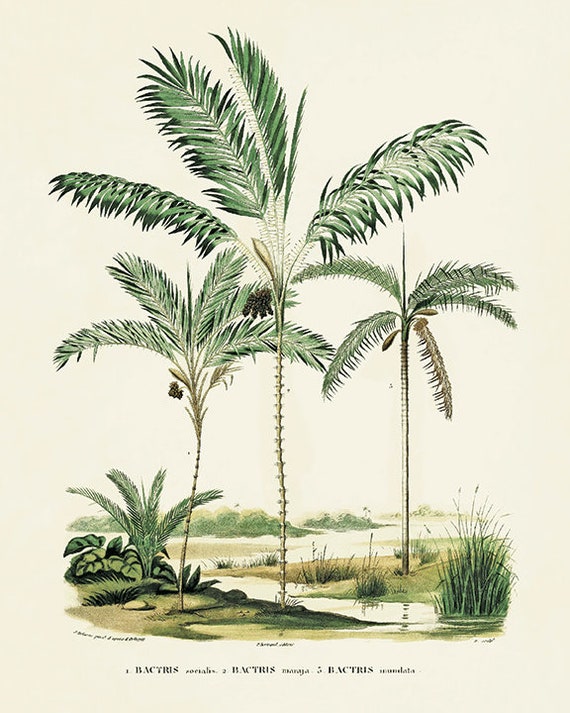The image is a detailed, hand-drawn illustration that appears to be from a nature guide, showcasing several types of palm trees alongside a body of water. The scene features various palm trees of different sizes and characteristics. The largest tree, located centrally, has a thin, slightly rough trunk adorned with small dark nuts at the top, and it appears to have thorns. On its left, a similar but smaller palm tree displays a smaller cluster of black nuts. To the right, another palm tree with a smooth trunk stands, displaying three larger clumps rather than a nut cluster. At the bottom, a ground palm tree is visible. The background includes scenic elements like a creek flanked by manicured lawns and rocks, brown patches of grass, green mountain ranges, and high palm trees with spiny accents and green leaves. Below the illustration, there is a small, hard-to-read description, with "Bacchus" being the first part of the scientific name. The entire setting, portrayed in portrait orientation, is complemented by a beige background.